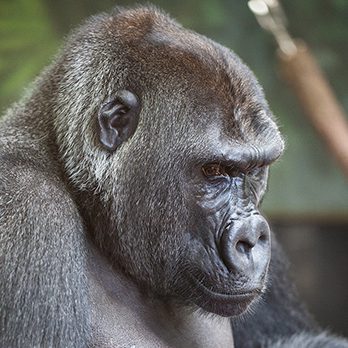A detailed colour photograph showcases the head and shoulders of a gorilla in its natural forest habitat. The gorilla, with a strikingly human-like face, is captured partly turned towards the right, almost engaged with the viewer. Its face is characterized by small, leathery black ears set high on the sides of its head and deep, sunken dark brown eyes beneath a heavy, prominent brow ridge. The nose is large and flat, giving a somewhat pig-like appearance compared to humans. Wrinkled, black leathery skin encases its face and mouth, which is closed and neatly tucked under the nose, flanked by sparse whiskers.

The gorilla's fur varies in texture and color: the head and back of the neck showcase a mix of grey and silver hairs, while the top of the head is tinged with brown. The chest hair appears shorter and more sparse, almost giving a leathery appearance. Under the combination of forest greens and indistinct background elements, the dominant silver and grey hues of its fur stand out, emphasizing the animal’s powerful and majestic presence. The precise object of the gorilla's gaze remains a mystery, adding an element of curiosity and contemplation to its vigilant posture.